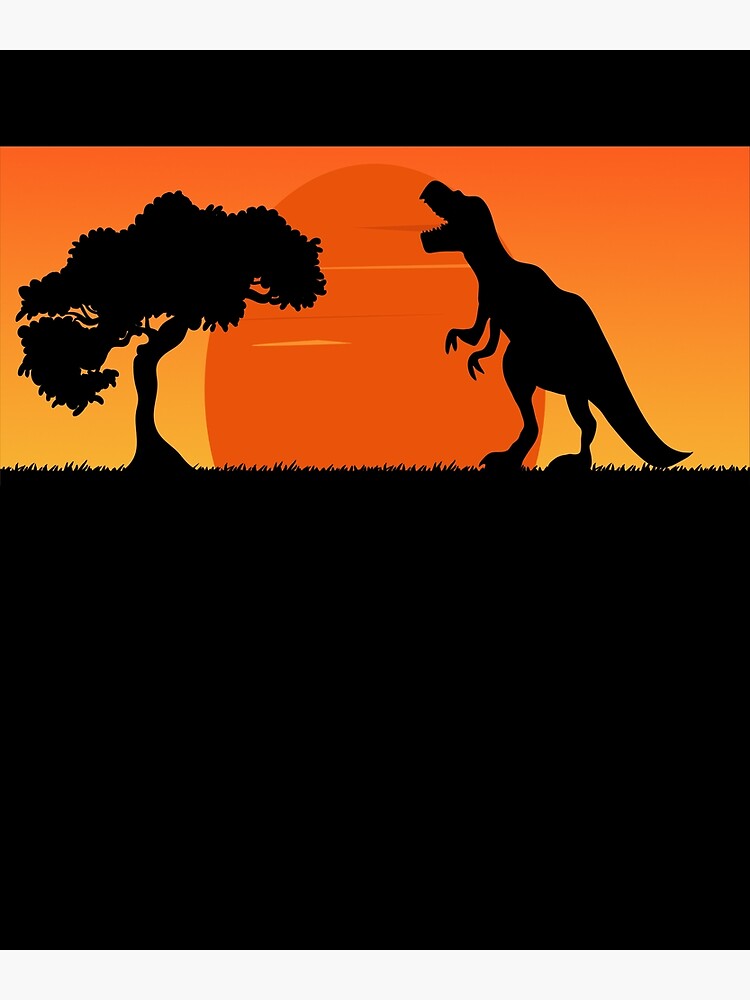This digitally created vertical image features a prehistoric scene with an orange backdrop that transitions to mustard yellow as it descends. Dominating the lower half of the image is a black expanse that represents the ground. Above this black base, the silhouettes of a roaring T-Rex and a blooming tree stand out starkly. The T-Rex, positioned on the right, is upright on its hind legs, facing left with its tail hanging down and its mouth wide open. The black silhouette of the tree, complete with branches and leaves or flowers, stands to the left of the dinosaur. Between them, a rounded orange sun with yellow stripes is nestled against the gradient sky. The scene is further detailed with an outline of black grass at the base, indicating that both the tree and the T-Rex are rooted in this ground area. The colors above the grass gradually shift from yellow to orange, resembling the hues of a sunset.